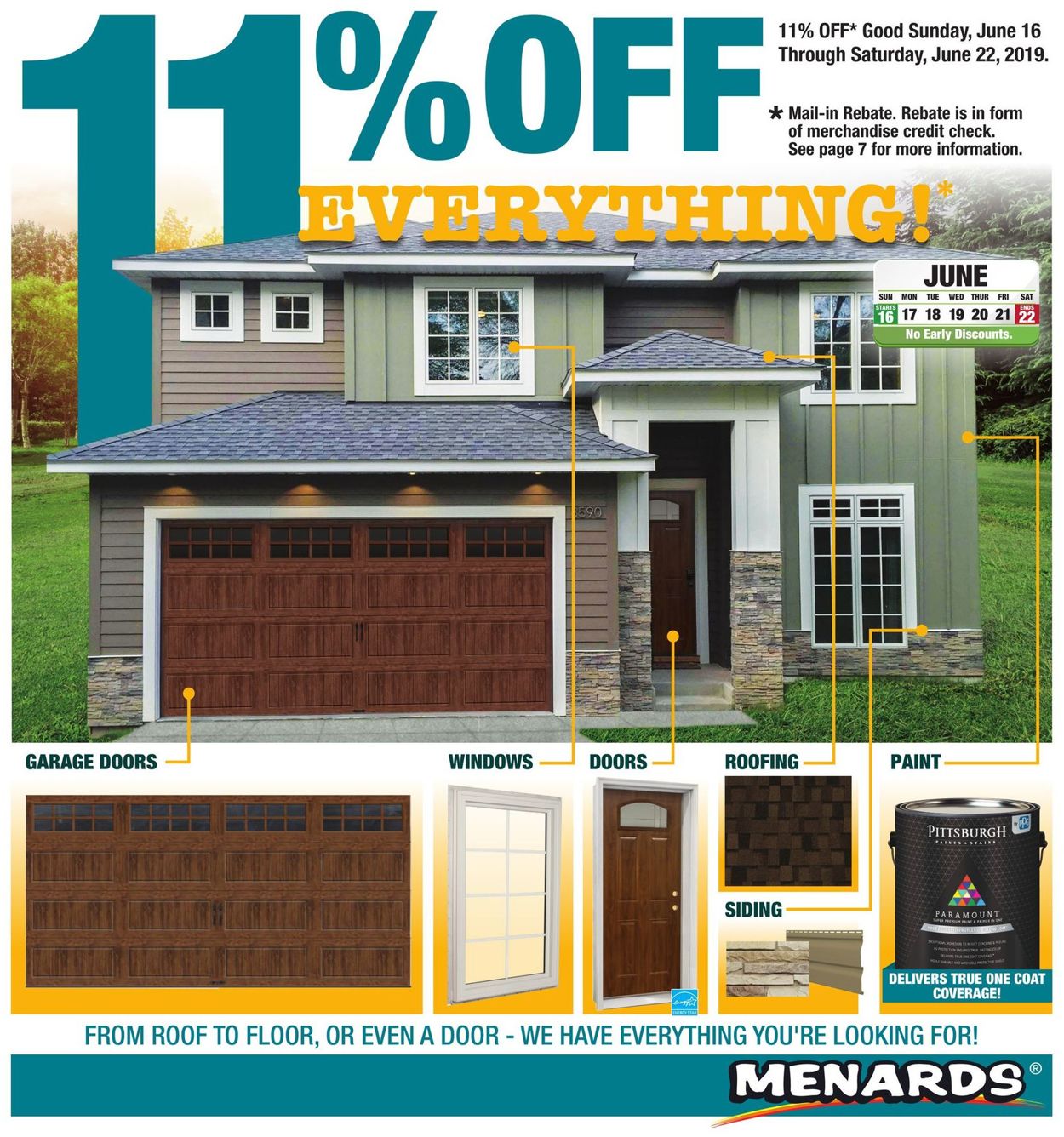Detailed Caption for the Menards Sales Flyer:

"Presenting the Menards sales flyer, prominently featuring a modern house with tan siding and white-framed windows, complemented by a white wooden garage door. At the top of the flyer, large bold text in blueprint style announces '11% OFF.' A yellow banner highlights the offer with 'EVERYTHING!' accompanied by an asterisk. In the upper right corner, black text specifies the sale period: 'Sunday, June 16th through Saturday, June 22nd, 2019,' noting that the 11% discount is available via a mail-in rebate, which will be issued as a merchandise check – further details can be found on page 7.

The lower section of the flyer showcases detailed, close-up images of the garage door, windows, front door, roofing, siding, and paint options. Beneath these images, set against a white background in blue text, the slogan reads: 'From roof to floor, or even a door, we have everything you're looking for.'

The flyer is encased in a blue border and branded on the right-hand side with 'Menards' in a playful Comic Sans script, outlined in black with a white fill. A registered trademark symbol appears in the upper right corner in blue, and a small yellow line underscores the Menards logo, concluding the design elements of the flyer."